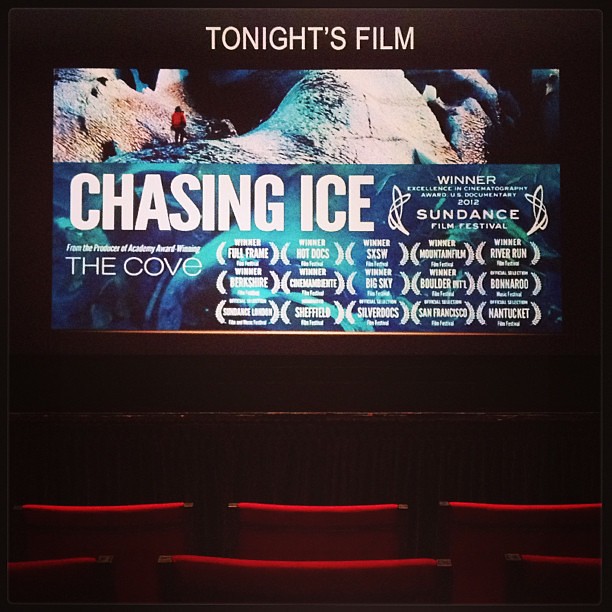In the dimly lit interior of a movie theater, rows of empty red chairs occupy the bottom of the image, leading up to a brightly illuminated screen at the top. The screen showcases a stunning poster for the film "Chasing Ice," featuring an image of a person in a red jacket standing on a vast iceberg, set against a backdrop of icy mountains. The headline on the screen reads "Tonight's Film," followed by the film's title, "Chasing Ice," in prominent white font. Below that, the text highlights the film's production by the Academy Award-winning producers of "The Cove." Accompanying the advertisement are numerous accolades, including Winner of the Excellence in Cinematography Award at the 2012 Sundance Film Festival, Full Frame, Berkshire, Hot Docs, Big Sky, and many more, which are listed across the image. The overall ambiance and detailed display of awards emphasize the film's critical acclaim and the theater's anticipation for this celebrated documentary.